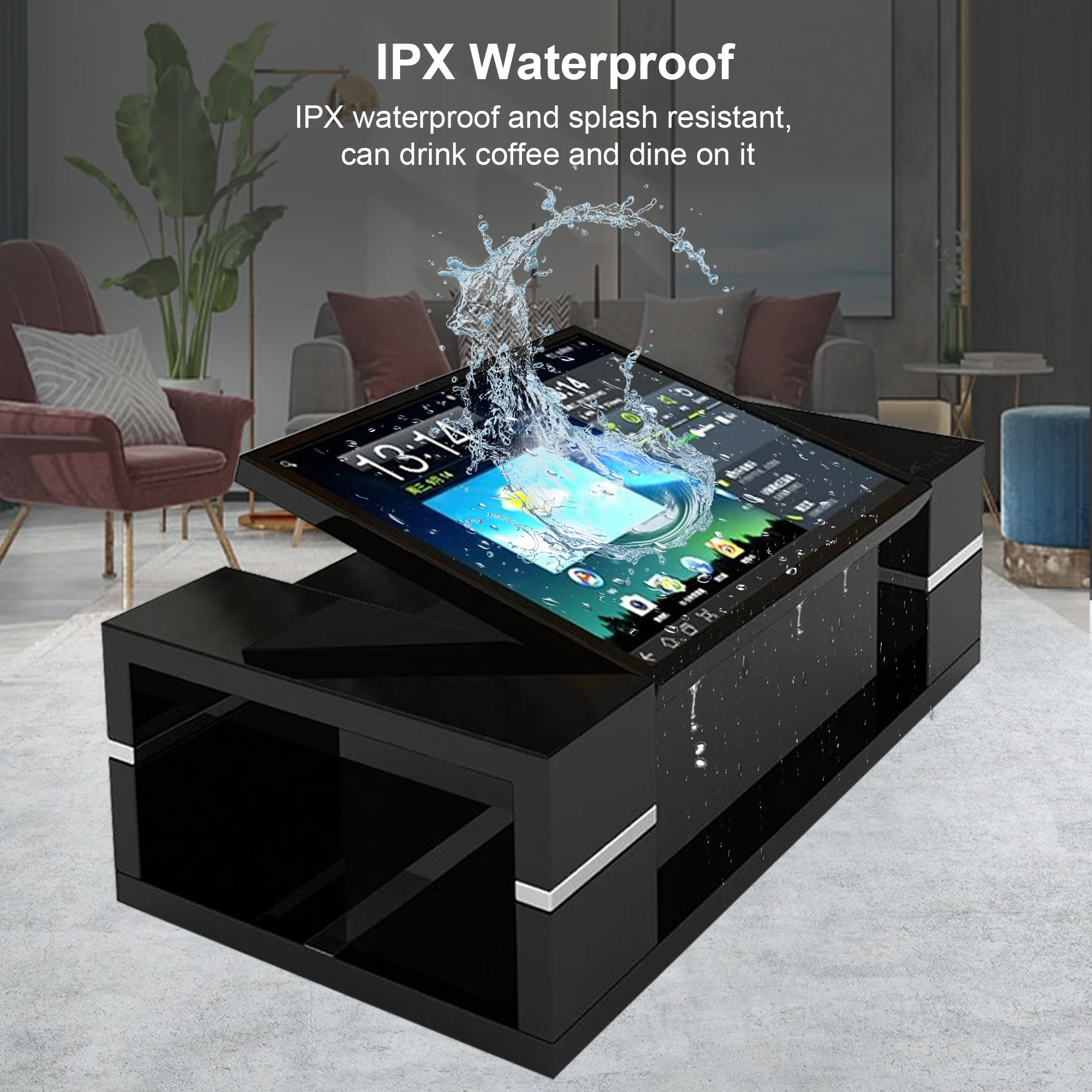The image appears to be an AI-generated advertisement highlighting a unique black coffee table that integrates a large, tiltable screen into its design. The table features silver accents and a tablet-like screen that covers most of its top surface. Text on the screen emphasizes its "IPX waterproof and splash-resistant" properties, suggesting that the table can endure spills, making it suitable for dining and drinking coffee. The screen displays the time as 13:14 and various icons, similar to those on a smartphone or laptop. Surrounding the table are chairs and a sofa, indicating it is placed in a living room setting. To underscore its water-resistant feature, the image includes a visual of a splash of water hitting the screen.